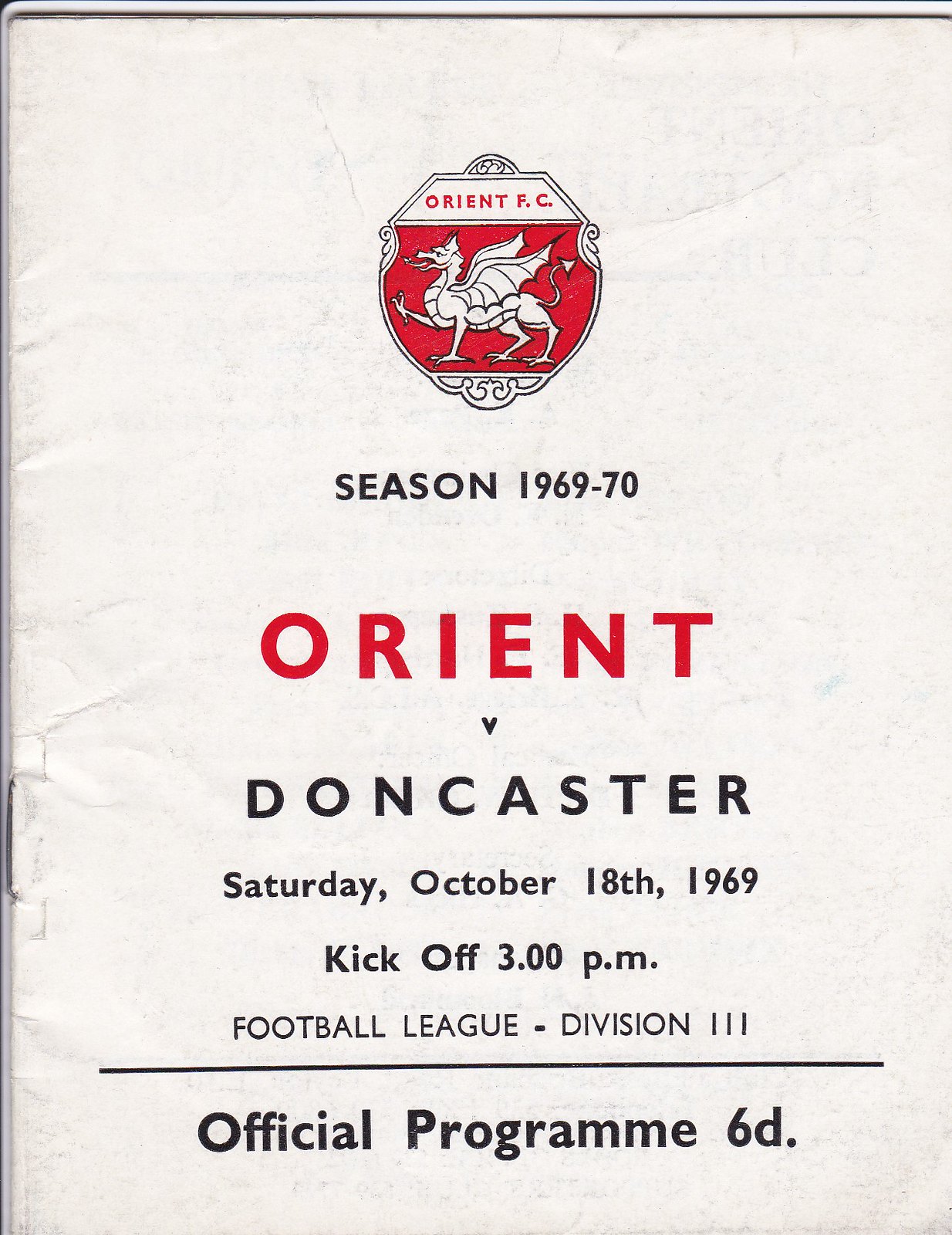The image depicts the cover of an old soccer program from the 1969-70 season, featuring a worn white paper background with visible staples on the left side holding the booklet together. At the top, there's a logo of a flying dragon within a symbol, labeled "Orient FC" on a red background. Below the emblem, the text "Season 1969-70" is written in black lettering. The prominent red text "Orient" appears beneath this, followed by "V. Doncaster" in black. Further down, the details of the match are listed: "Saturday, October 18, 1969. Kickoff, 3 p.m. Football League, Division III." A horizontal black line separates this information from "Official Program 6D" at the bottom. The paper has signs of age, with black stains and creases. This appears to be the cover of a multi-page booklet.